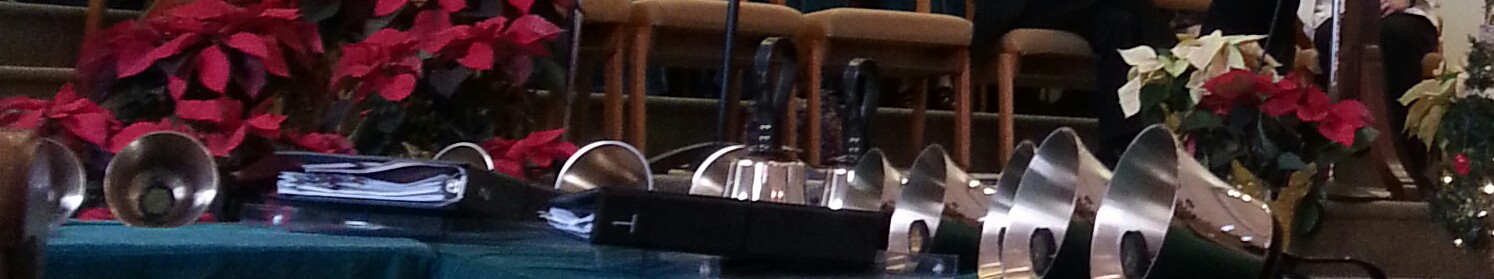This color photograph is a horizontal, rectangular image showcasing the bottom of a stage decorated for what appears to be a Christmas setting. The left side of the stage is adorned with vibrant red poinsettia flowers, while the right side features a mix of red and white poinsettias, accompanied by lush green leaves. In the center of the stage, there are several brown chairs with thin brown legs. Positioned in a neat line across the front of the stage are numerous large silver bells with black handles, reminiscent of those seen during Christmas. Scattered in the middle of the image are two black binders, each brimming with thick stacks of white paper. The lower left-hand corner of the photo reveals a medium blue table, behind which stands a brown wood cabinet with three sections and glass doors.